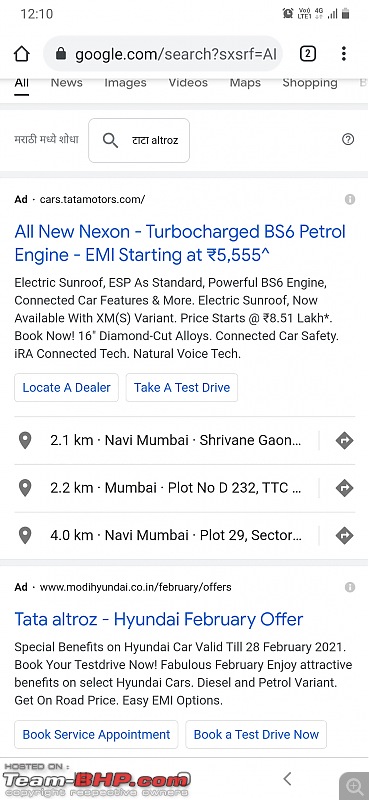The image is a screenshot of a mobile device displaying a Google search results page. The address bar at the top shows "google.com." Below the address bar, there's a navigation menu with tabs labeled "All," "News," "Images," "Videos," "Maps," and "Shopping," with two of the tabs presented in a different language. The top search result features an advertisement for Tata Motors at "cars.tatamotors.com." The ad promotes the all-new Nexon, highlighting its turbocharged BS6 petrol engine with EMI starting at 5,555 rupees and upwards. Below the ad, some of the car's features are listed. The page also displays three locations relevant to the search query. At the bottom of the screenshot, another ad mentions the Tata Altroz and a February offer from Hyundai, with the source website "team-bhp.com" listed in the bottom left corner.